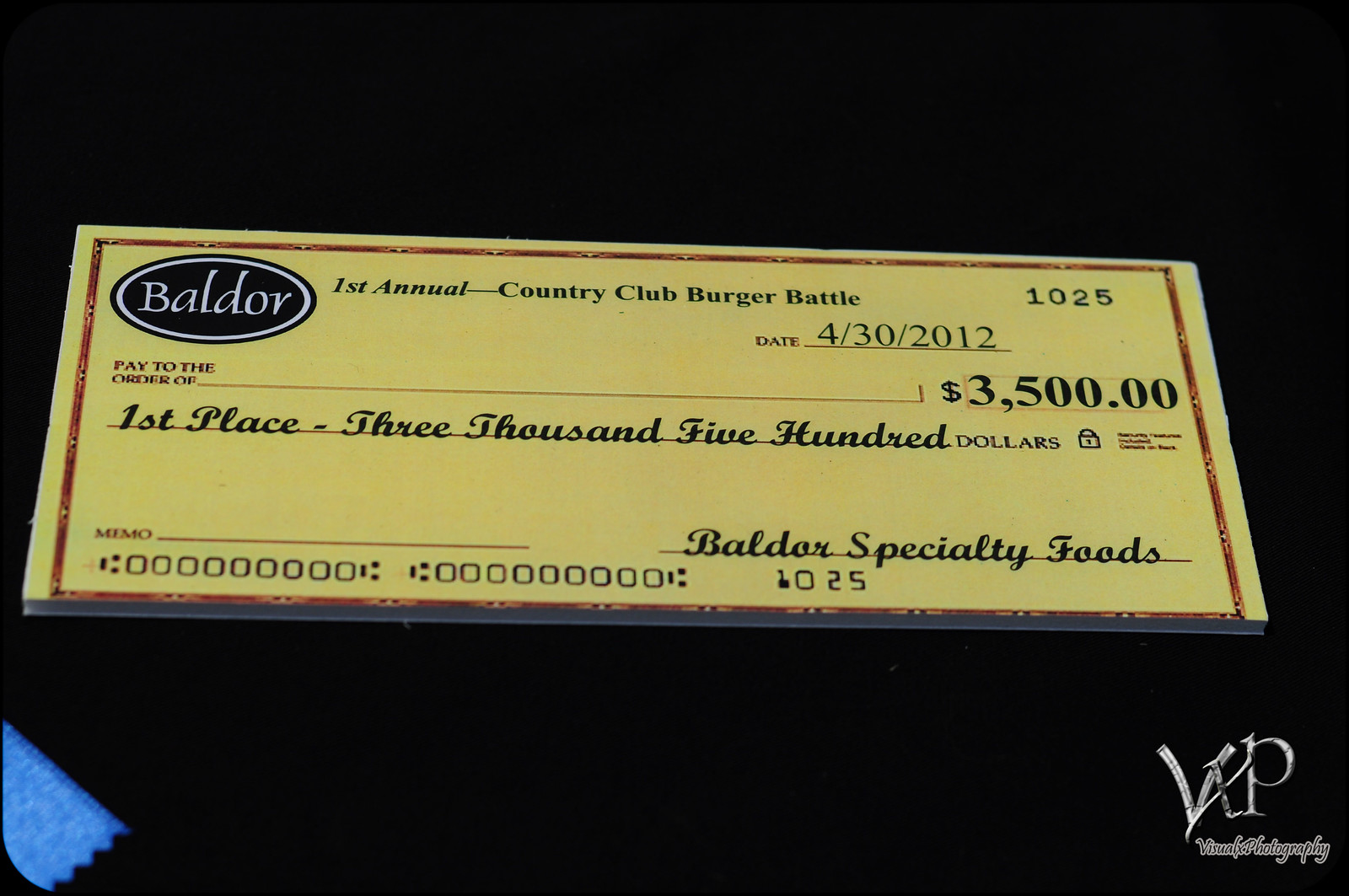The image features a yellow check against a pure black background, angled slightly downward. The check is associated with the "First Annual Country Club Burger Battle" and features the Baldor Specialty Foods logo prominently in the top left corner. The logo consists of the name 'Baldor' in white text within a black oval, outlined in white. The check is dated 4-30-2012 and is designated as check number 1025. It is made out for $3,500, both in numerals and written out as "First Place $3,500." The check has a blank memo line and is not addressed to a specific recipient. The signature at the bottom confirms it is from Baldor Specialty Foods. Additionally, there is brand text "VXP" in the bottom right corner of the check.